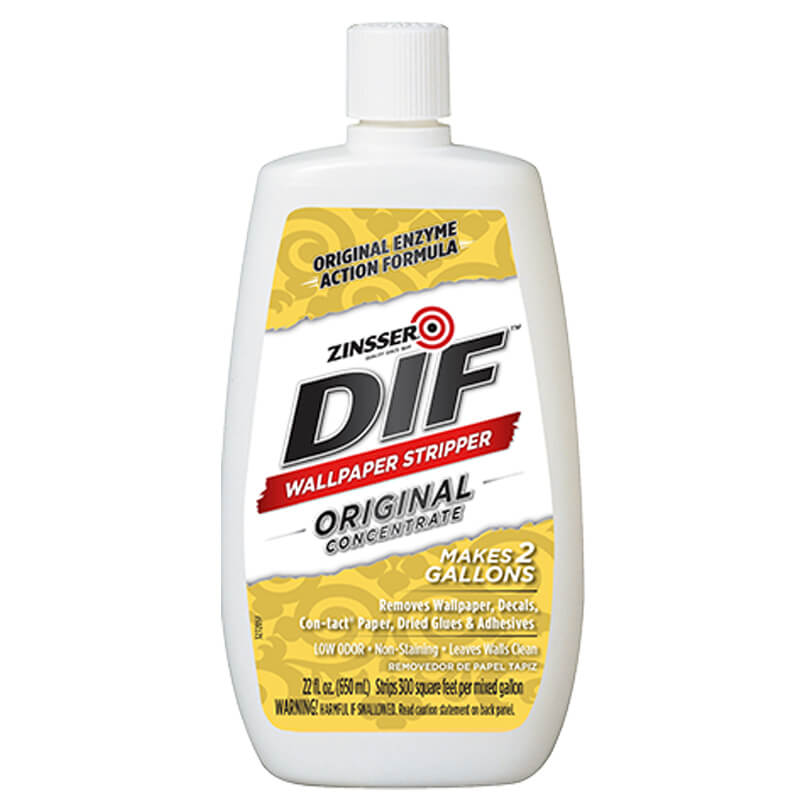This image features a detailed photograph of a white plastic bottle of Zinsser DIF Wallpaper Stripper, standing on a plain white background. The bottle is approximately five inches tall and slightly round at the bottom, with a white twist cap that is about three-quarters of an inch high and wide. The bottle's body gradually expands from about one and a half inches wide at the top to two to two and a half inches at its base.

The label on the bottle is predominantly yellow and white with elements of red and black. The top section of the label is yellow with light gray circles and features black text that reads, "Original Enzyme Action Formula." Below this, a diagonal white stripe displays the product name, "Zinsser DIF," in bold black print, followed by "Original Concentrate" underneath in smaller text. The next segment showcases a red banner with white text proclaiming it as a "Wallpaper Stripper."

Further down, the yellow background reappears and provides key details in white text. It states that the formula, when mixed, makes two gallons and is effective for removing wallpaper, decals, contact paper, dried glues, and adhesives. Additional attributes include "Low Odor, Non-Staining, Leaves Walls Clean." The capacity of the bottle is 22 fluid ounces or 650 milliliters, with efficacy speculated at stripping 300 square feet per mixed gallon.

At the very bottom of the label, black text provides cautionary information, noting that the product is harmful if swallowed and advises the user to read the warning section on the back panel.

Overall, the bottle's design reflects a functional and informative aesthetic suited for its utility purpose.